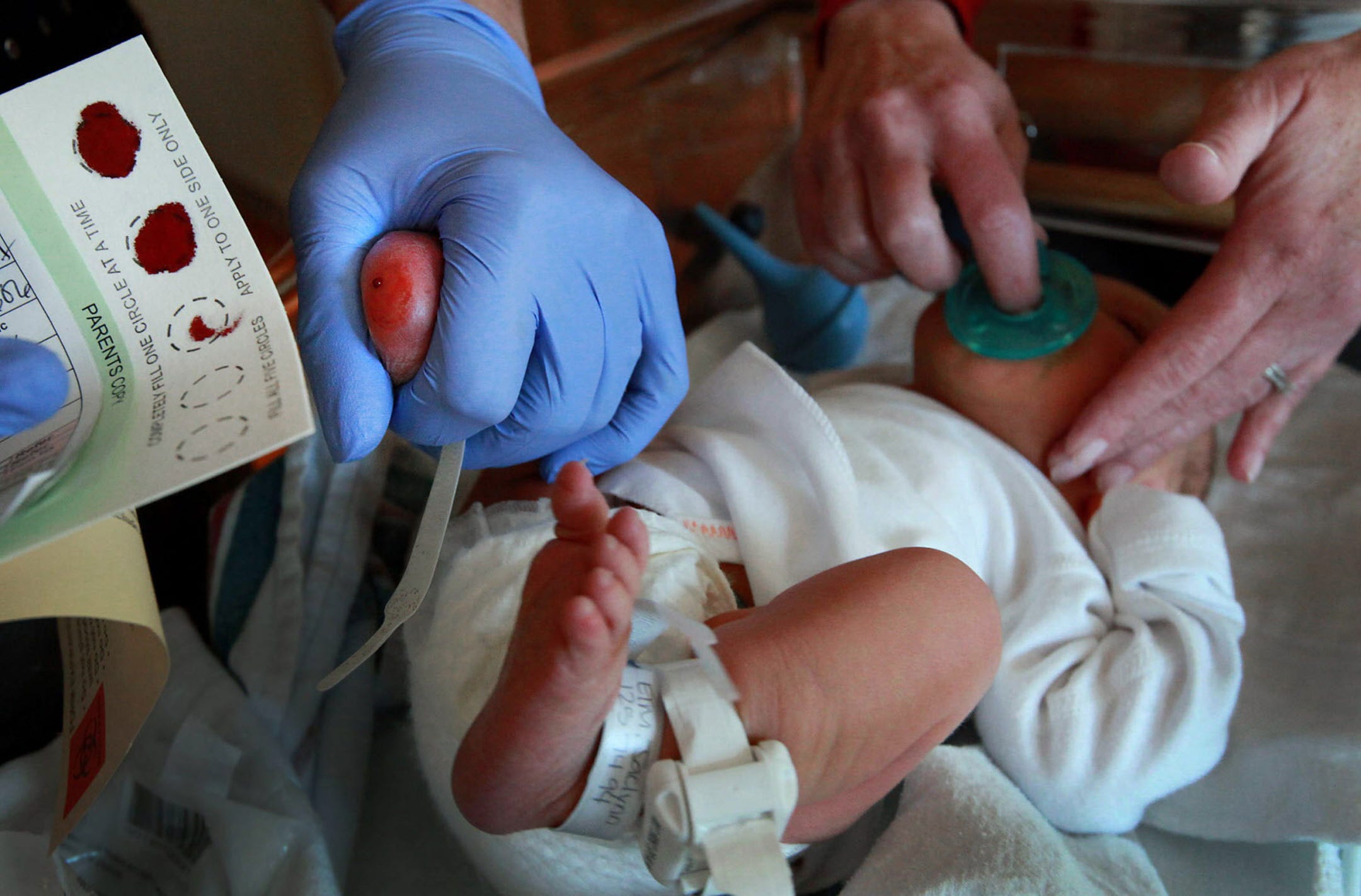The image depicts a very small baby undergoing a medical treatment, likely a blood draw, in a hospital setting. The baby, wearing an unbuckled white onesie and a small diaper with a security tag labeled "Jacqueline Elm," has its legs curled up. A person with a female's hand gently touches the baby’s cheek while holding a green pacifier in its mouth. Alongside the baby's head rests a blue suction tool. Another individual, possibly a nurse or doctor, donning light blue medical gloves, is handling the baby's foot, which appears to have a small drop of blood and is slightly red from a prick. This same person is holding a piece of paper that has circular blood stains and instructions visible, suggesting it's a blood sample collection card. The card also bears text that reads "parents" and "fill one circle at a time" along with "apply to one side only," indicating the procedure's steps.